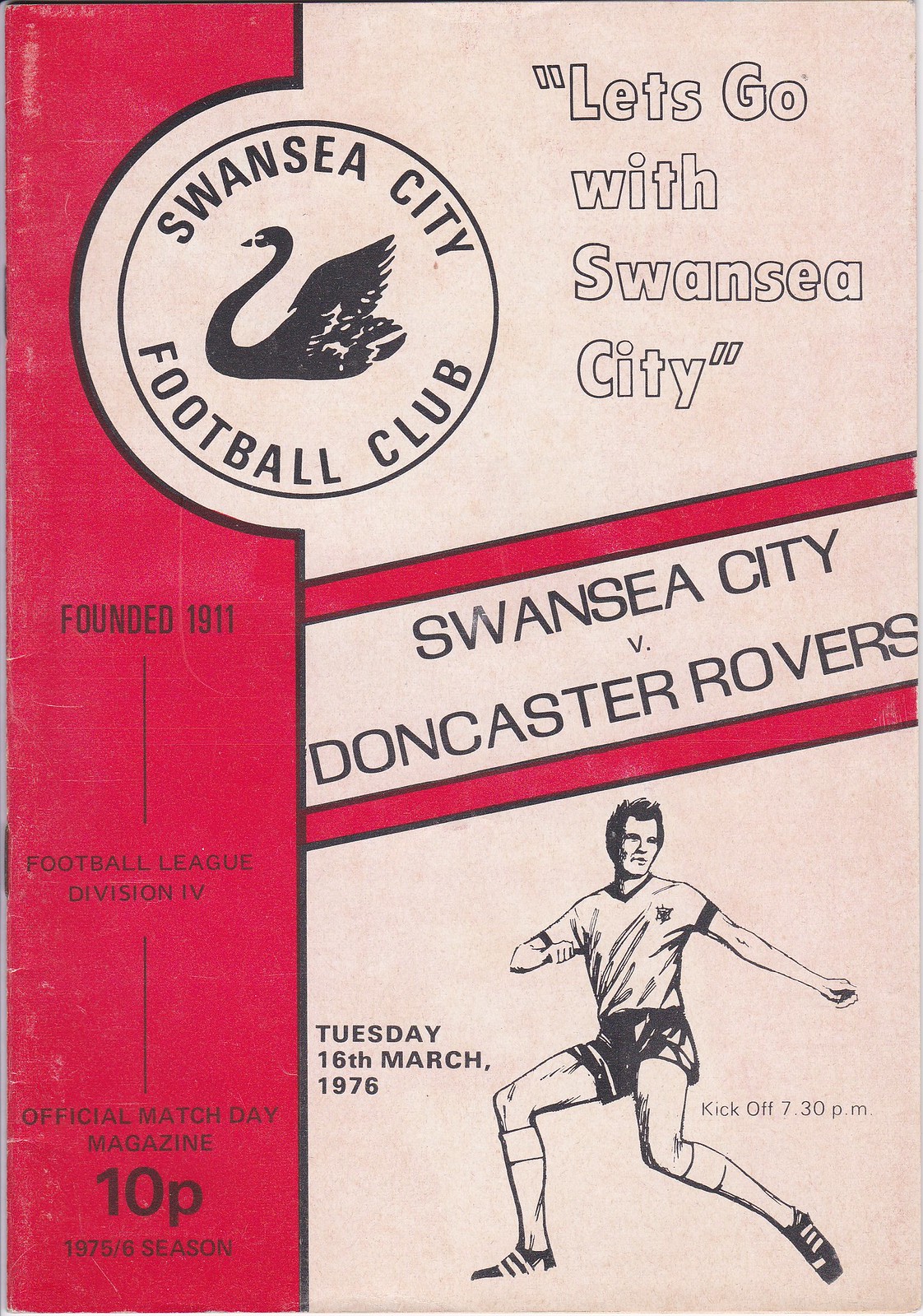This is a photograph of a vintage football program cover for a match between Swansea City and Doncaster Rovers. The left half of the cover is red, and the right half is a peach color. At the top, it features the text "Let's go with Swansea City" adjacent to a circular logo with a swan in the middle that reads "Swansea City Football Club." Below that, centrally positioned, is a banner stating "Swansea City versus Doncaster Rovers." Underneath the banner, there is a detailed line drawing of a football player in motion. On the right side of the player, the text "Kickoff 7.30 PM" is displayed. On the left side, it reads "Tuesday 16th March 1976." Further details include the text under the swan logo on the red side: "Founded 1911, Football League Division 4, Official Match Day Magazine, 10-P, 1975-76 season."